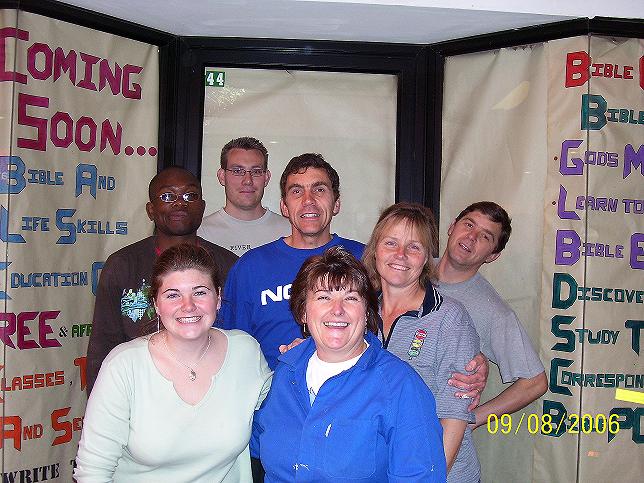In this photograph dated 09-08-2006, seven people of varied ages, primarily in their 30s except for a woman around 50, pose in front of a black door with a cream-colored covering. The group consists of four men and three women, with the men including one African-American gentleman with glasses in a brown sweatshirt, a man in a blue t-shirt, a man in a gray t-shirt, and a short blonde-haired man with glasses in a beige t-shirt. The women, two of whom are at the forefront with their arms wrapped around each other, are all smiling or looking at the camera, with a couple showing neutral expressions. The background features angled walls adorned with plastic signs in vibrant colors like hot pink, light blue, orange, purple, red, and black. The left sign reads, "Coming Soon, Bible and Life Skills, Education, Free Classes," while the right sign shows fragmented words like "Bible," "Discover," "Study," and "Correspondence."